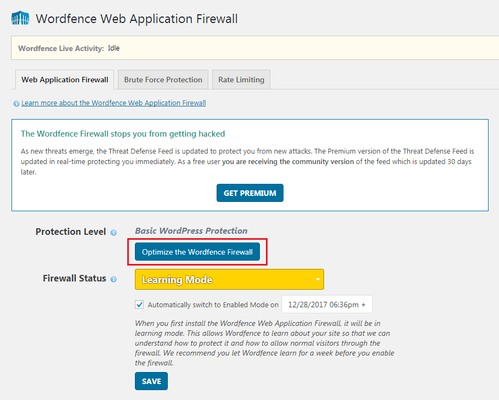This image is a cropped screenshot of the WordFence Web Application Firewall interface, featuring a grey background. At the top of the interface, there is a blue fence icon followed by the text "WordFence Web Application Firewall". Directly beneath this header is a substantial text box with a yellow background, containing the small grey text "WordFence Live Activity Idle" on the left side.

Below the yellow text box, there are three tabs aligned horizontally: "Web Application Firewall" (highlighted as selected), "Brute Force Protection," and "Rate Limiting." Under the selected Web Application Firewall tab, there's an info icon leading to a hyperlink titled "Learn more about the WordFence Web Application Firewall" written in underlined blue text.

Underneath this section lies a large white box with a blue outline containing the message "The WordFence Firewall stops you from getting hacked." Directly beneath this message is a brief description, and, centered at the bottom of the box, the text "Get Premium" is displayed.

Outside the white box, aligned to the left and below, the words "Protection Level" are presented, with "Basic WordPress Protection" shown to the right. Beneath this descriptor is a blue button labeled "Optimize the WordFence Firewall," which is outlined in a red box to draw attention. Further down, the text "Firewall Status" appears with a selectable drop-down box set to "Learning Mode," highlighted in yellow. This drop-down box is meant to indicate the current operational mode of the firewall.